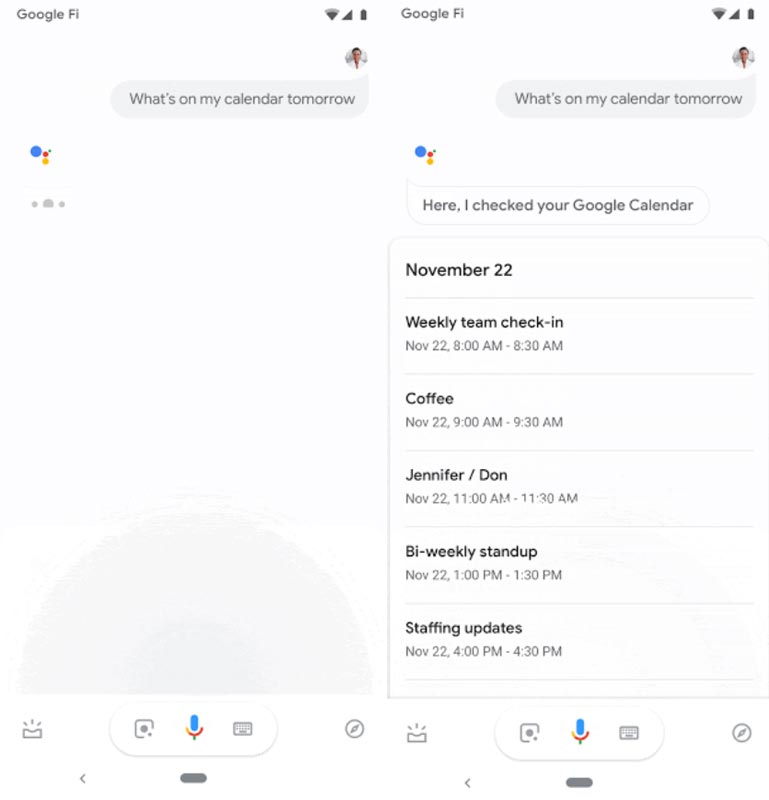The image consists of two screenshots displaying the Google Fi Wi-Fi calling interface.

In the left screenshot:
- The top left corner features the "Google Fi" label in a gray font.
- To the right, icons for Wi-Fi, data, and battery status are visible.
- Directly below, a rounded user icon shows a man with dark hair wearing a white shirt.
- A light gray message bubble features gray text that says, "What's on my calendar tomorrow?" followed by the Google Assistant logo. Three dots indicate that a response is being typed.
- At the bottom left, a gray icon resembling a rectangle with three lines emanating from a dip in the middle is visible. 
- An oval area with a shadowed gray border contains a camera icon, a microphone icon, a keyboard icon, and a circular icon with a compass symbol, suggesting web access through Safari.

In the right screenshot:
- Similar to the left, the user icon is again at the top right.
- The Google Assistant response is displayed in a white text bubble. It reads, "Here, I checked your Google calendar." 
- Below, in bold text, "November 22nd" is given, followed by a divider. 
- A detailed schedule includes "Weekly Team Check-In" in bold with "NOV 22, 8:00 AM – 8:30 AM" in light gray beneath it.
- Another gray divider follows, leading to "Coffee" in bold black text, with "9:00 AM – 9:30 AM" listed below in small gray lettering.